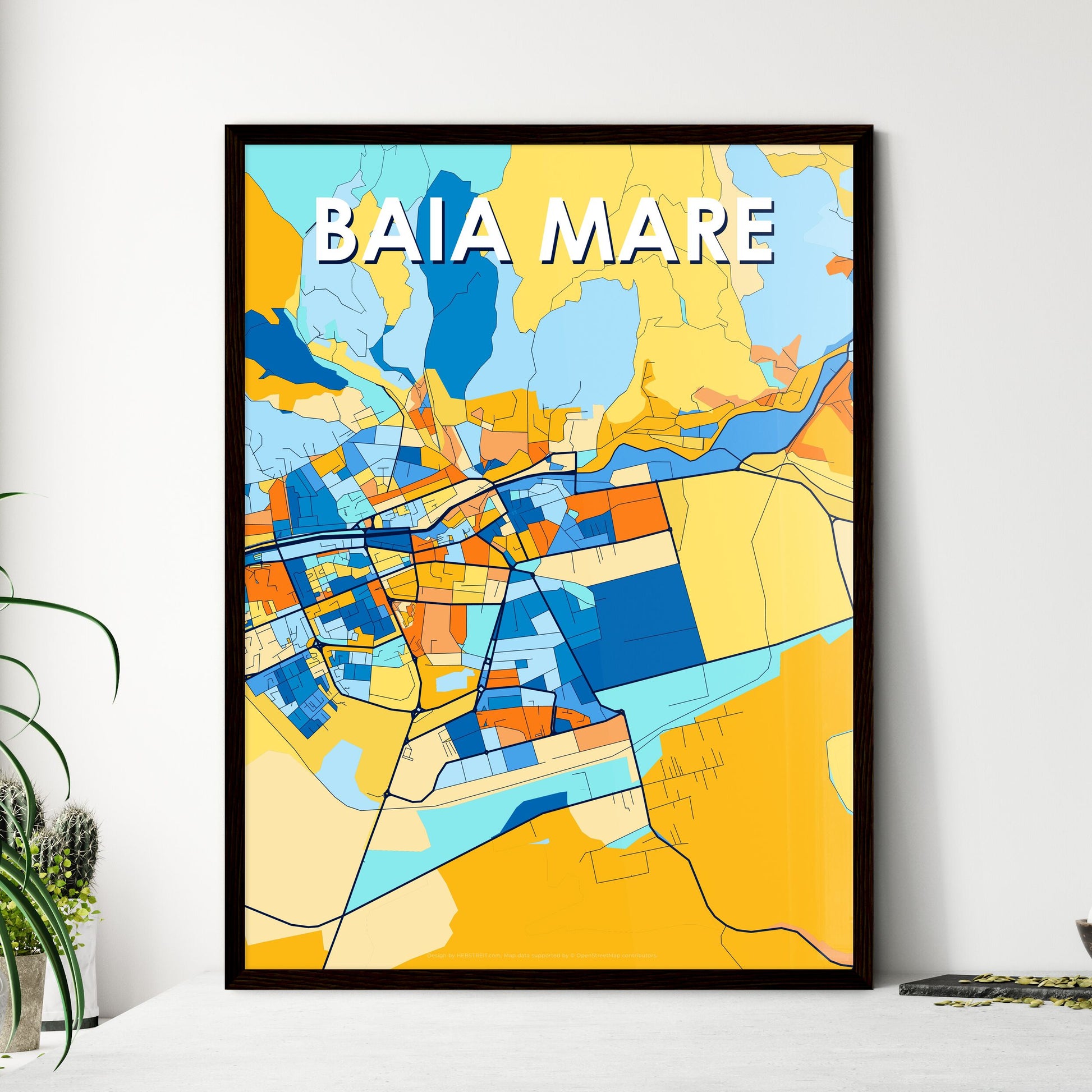This image showcases a poster titled "BAIA MARE" in uppercase white letters at the top, prominently displayed within a thin black frame. The poster, mounted on a white wall, features a map with a colorful palette that includes various shades of blue, yellow, orange, and green, with black lines representing roads. The bottom left corner of the image reveals green-leaved foliage, potentially including a cactus, while the bottom right depicts a gray and green flat object that resembles moss or pistachios, possibly part of an artwork or a decorative piece.